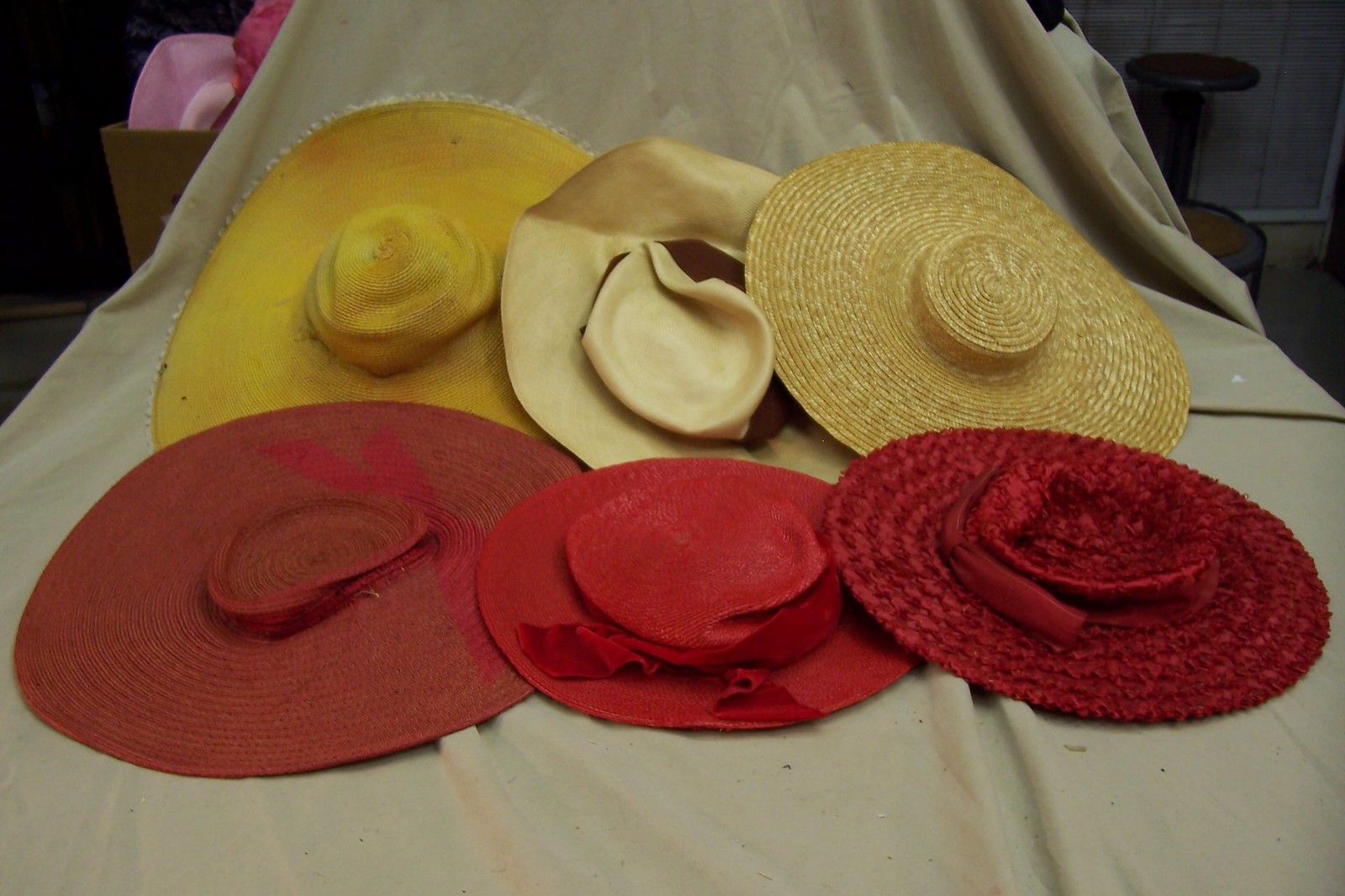The color photograph, taken under low, artificial lighting with a yellow tint, showcases six large sun hats laid out on a tan, dark beige, cyan-colored sheet. The hats are arranged in two rows of three each. In the front row, there are three red hats of varying sizes and details: the leftmost hat has a very wide and thin brim; the middle hat is smaller with some height and features a red velvet-like scarf or ribbon around it; and the rightmost is a textured red hat with a red bow. The back row consists of three hats in shades of yellow and tan: the leftmost hat is bright yellow with a wide brim and frayed edges, showing significant wear; the middle hat is a light tan color and appears heavily wrinkled or crushed; and the rightmost hat is a yellowy tan, straw or wicker hat with a distinguished pattern of lines, making it pliable and bendable. These hats, contrasting in colors and textures, display significant wear or aging, giving them a distinct character in the image.